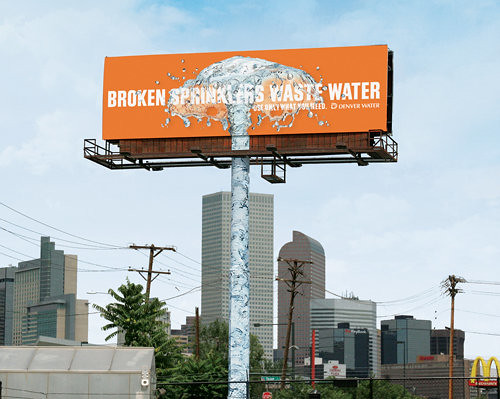The image depicts a striking cityscape featuring a high-up, orange billboard that prominently reads "Broken Sprinklers Waste Water" in white text. Positioned centrally, the billboard includes a dynamic design of water erupting, which seamlessly extends down the pole supporting the sign. This clever artistic choice makes it appear as if the water is shooting up from the ground, through the pole, and cascading onto the billboard itself, creating a visually arresting effect akin to a geyser. The billboard is equipped with a metal railing and scaffolding for maintenance access.

In the background, we see a mix of high-rise and lower-profile buildings, including a typical square office building and more intricately designed structures, suggesting a bustling urban environment. A McDonald's sign is visible amidst this cityscape, adding a touch of familiar commercialism. Fluffy white clouds scattered across a light blue sky add a sense of depth and atmosphere to the image. In the foreground, there are some trees and what appears to be part of a residential area, possibly a greenhouse. Power lines and telephone poles intersect through the scene, tying together the urban and residential elements. The billboard also hints at a local context by including "Denver Water" in smaller text, suggesting the location is Denver, Colorado.